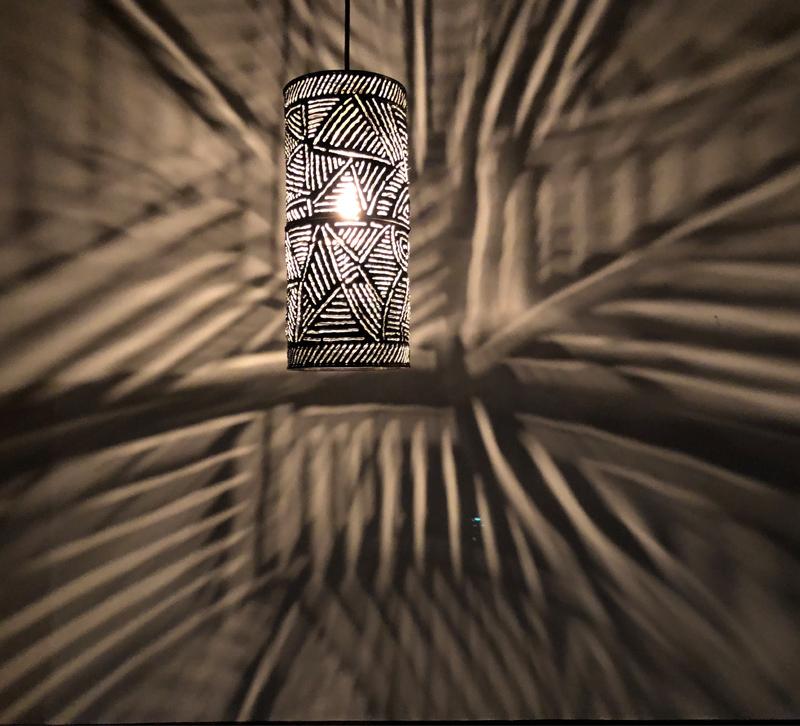This image captures an intricately designed ceiling lamp suspended by a black cord. The lamp itself is cylindrical and features a series of intricate, tribal-like engravings and cutouts that allow light to shine through. These cutouts create a mesmerizing pattern of lines and shapes, casting shadows and light onto the surrounding walls. The backdrop appears slightly hazy and blurred, predominantly in shades of beige and brown, with stick-like shadows contributing to a cathedral or hut-like ambiance. This detailed interplay of light and shadow gives the entire scene a deep, almost ethereal quality. The lamp's illuminated design not only transforms the space but also reflects off nearby surfaces, enhancing the captivating visual effect.